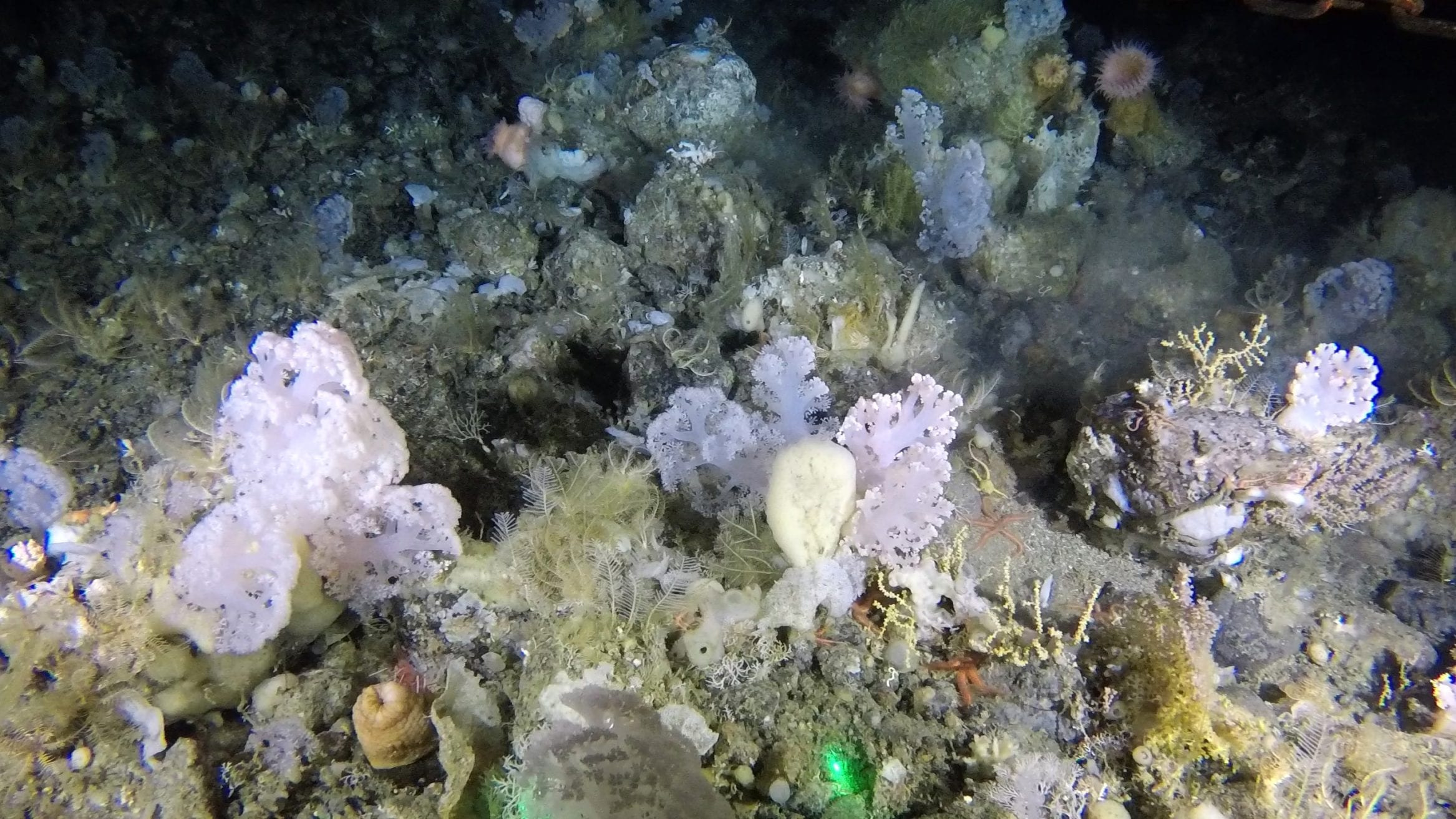This detailed underwater scene, depicted in a horizontal watercolor painting, portrays a vibrant coral reef arrayed with diverse hues and textures. The foreground bursts with lively colors, featuring corals in shades of pink, lavender, cream, and brown, interspersed with sea sponges of various colors, including pink and yellow. Sea sponges, round in shape, and yellow grass-like sprouts jutting from some of the corals add to the rich tapestry of marine life. Though devoid of fish, the reef features moss and potential camouflaged animals, blending seamlessly with the appearance of rocks on the ocean floor. The painting showcases a play of light, with the foreground illuminated brightly, transitioning to a darker background that signifies the deeper ocean, emphasizing the gradient from the ocean’s light-filled upper layers to its shadowy depths.